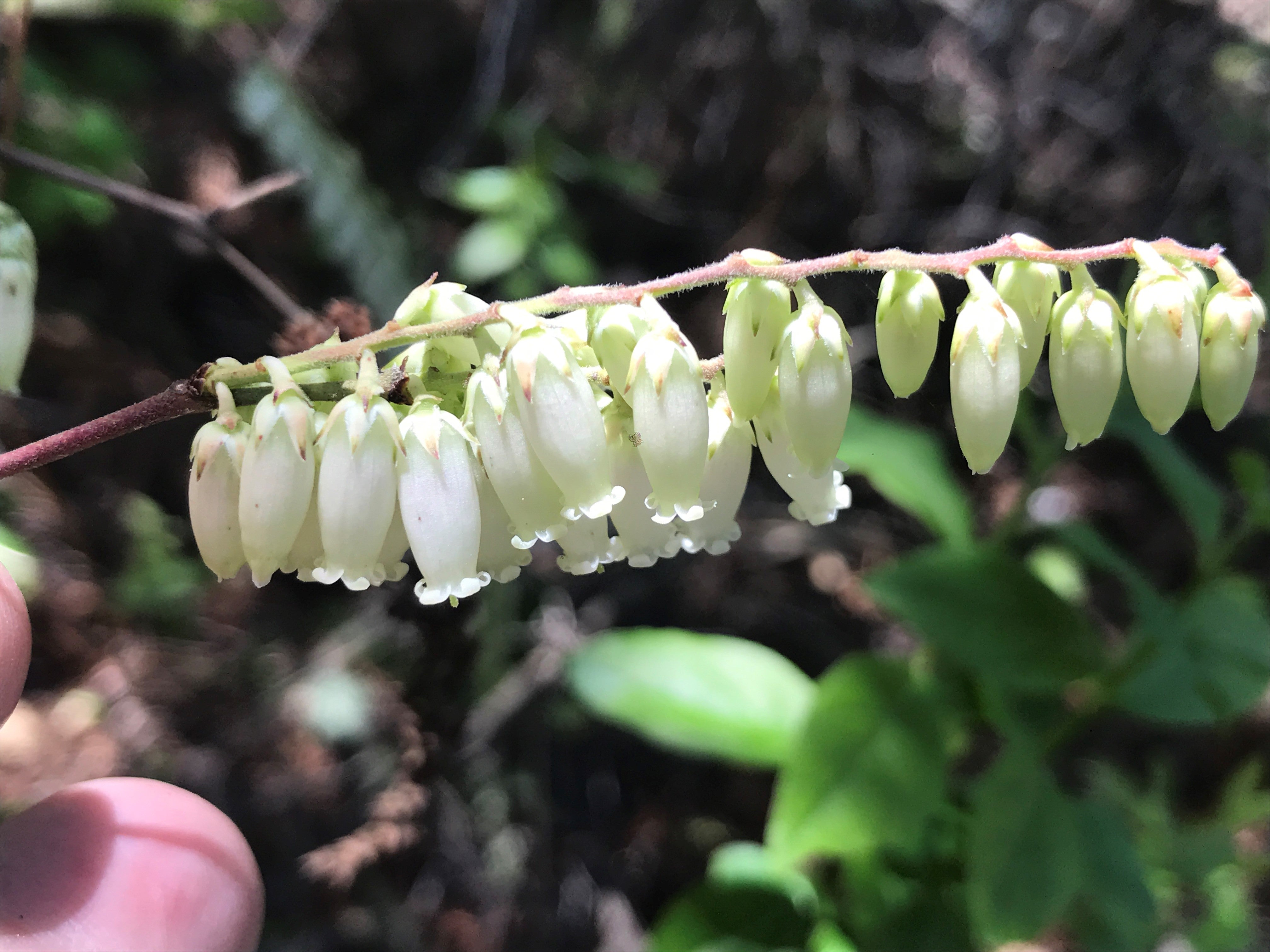The image captures a serene natural scene, focusing closely on a plant. On the right-hand side of the photograph, the bottom section is lush with green leaves. As the viewer's gaze moves upward, the image becomes increasingly blurry, but earthy brown tones stand out. In the bottom left-hand corner of the frame, a hand gently holds a leaf, revealing the tips of two fingers. The plant's stem begins as a rich brown and gradually transitions to a nearly white hue. On this lighter part of the stem, clusters of tiny, unopened flowers dangle delicately. The petals of these nascent blooms are primarily white but feature subtle light green hues where they connect to the stem. The overall scene exudes a peaceful moment in nature, capturing the intricate details and evolving colors of the plant.